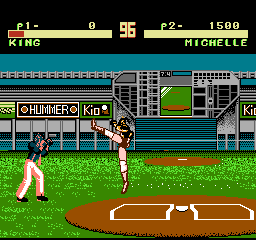The image depicts a retro arcade video game set within a baseball stadium. The game interface features player designations "P1: King" and "P2: Miguel," with score indicators showing "96" for P1 and "1500" for P2. The scene is centered around a baseball field, including a prominently visible brown pitcher's mound with a home plate. Two characters are engaged in combat on the field: one character, dressed in a black uniform, is executing a high karate kick, while the other, wearing pink pants and a blue shirt, adopts a defensive stance with fists raised in a boxing pose. Above the action, a sign reads "Hummer Keough," adding to the nostalgic atmosphere of the stadium setting. The overall aesthetic evokes the charm and simplicity of classic arcade games.